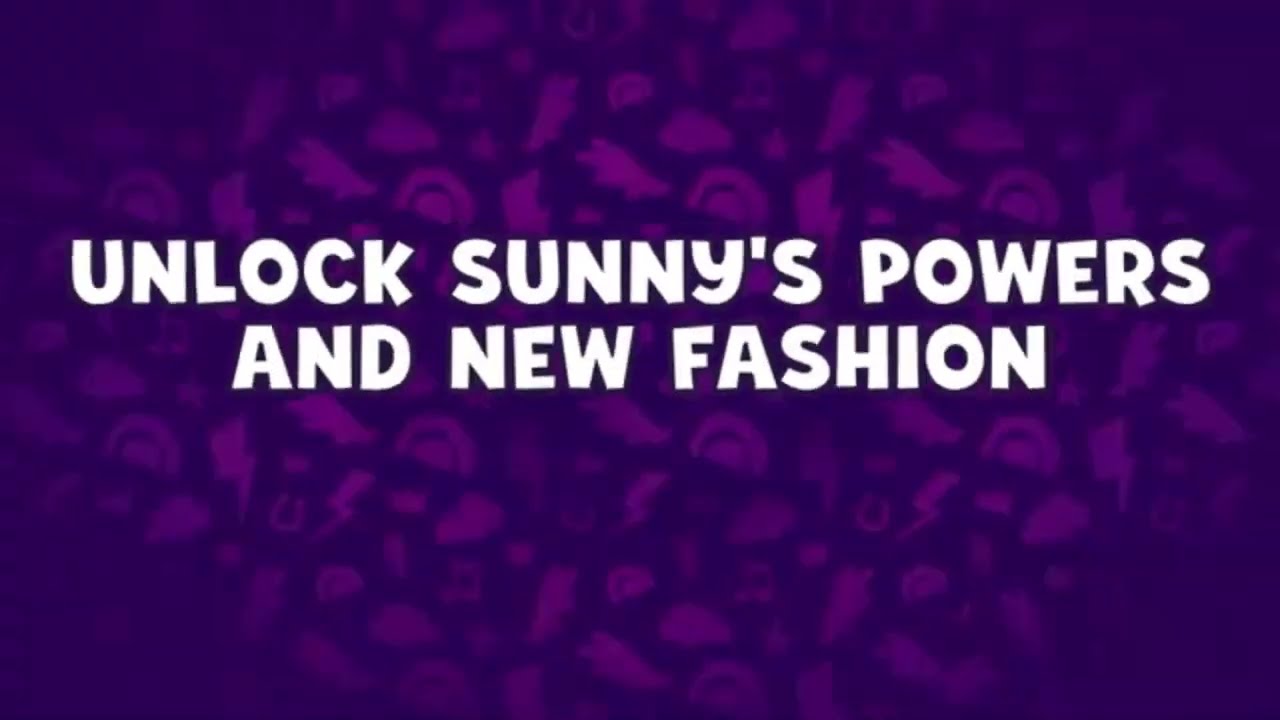The image showcases a landscape-oriented rectangle with a predominantly dark purple background adorned with various lighter purple shapes. These shapes include lightning bolts, rainbows, horseshoes, leaves, squares, and a few indefinite ones like a sun with a ring and a cloud-like figure. Centered near the top of the image, in bubbly, white, all-capital letters, is the text "UNLOCK SUNNY'S POWERS," followed by "AND NEW FASHION" on a new line. This fun and feminine text is not justified to the left or right but is centered, contributing to a balanced and lively design.